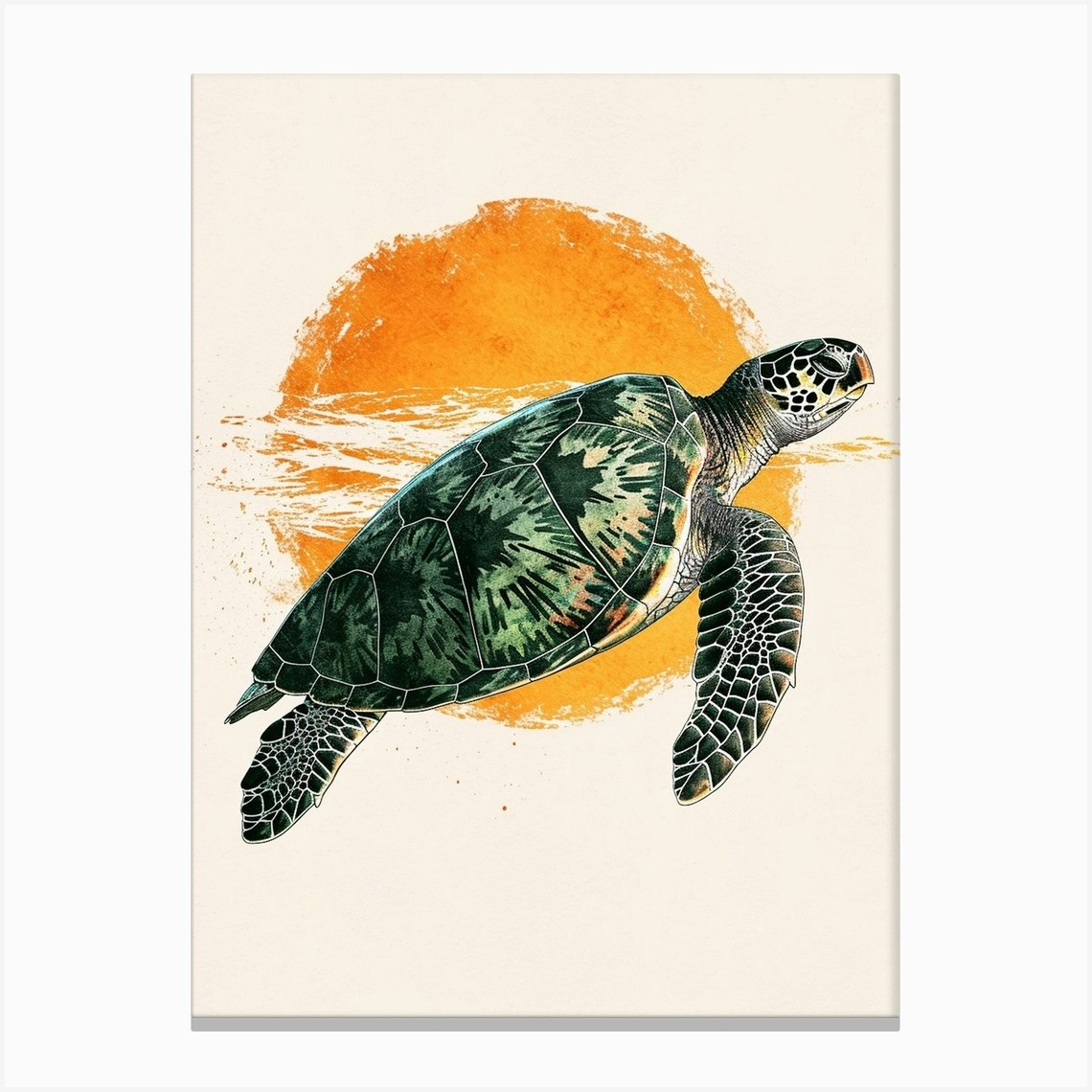The detailed and combined caption for the image is as follows:

The image showcases a meticulously painted sea turtle, set against a plain cream background which gives an impression of a white canvas. Central to the composition is a radiant orange-yellow sun half-submerged in crystal clear water, its reflection creating a near-perfect circle that suggests waves. The sea turtle, swimming gracefully to the right with its flippers spread wide, is intricately detailed. Its shell exhibits a rich mosaic of black, green, orange, yellow, and tan hues. The turtle's legs have a scaly black and white pattern, while its head, adorned with black dots, features a yellow face and an orange beak-like mouth. The overall scene captures a serene moment, illustrating the turtle ascending from the water with a sense of dynamic motion.